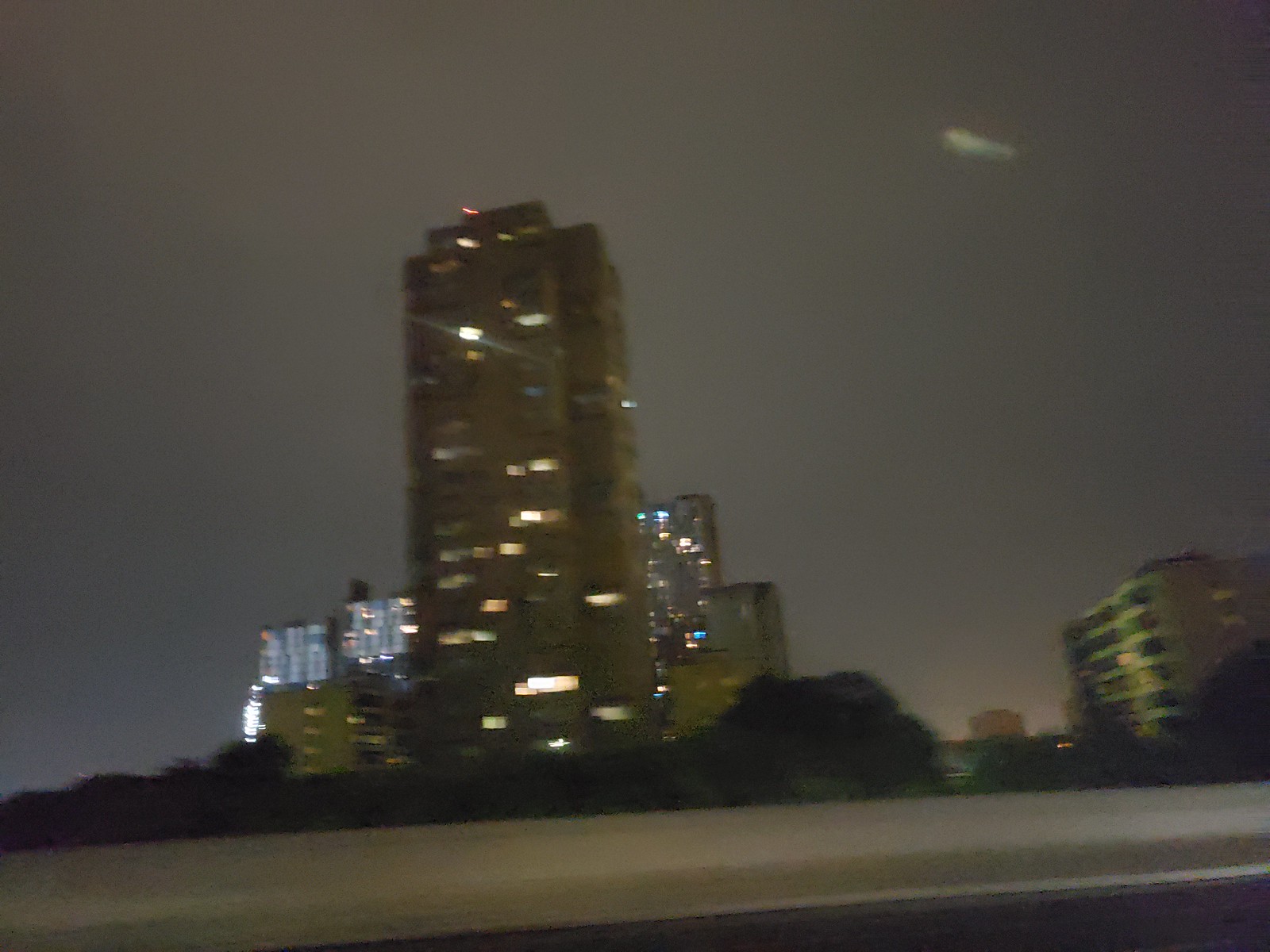Captured from a moving vehicle at night, this photograph features a blurred cityscape viewed through the side window. In the foreground, the slanted side rail of a highway hints at the vehicle's motion. The night sky is a deep black, devoid of stars except for a faint tiny cloud. Dominating the center is a tall building, likely around 14 to 20 stories high, with a mix of lit and unlit windows, possibly an office building or hotel. Surrounding it are several shorter buildings, varying from dark to dimly lit, with a particularly noticeable five-story building to the right. In the background, silhouettes of bushes and trees can be faintly seen, adding layers to the urban scenery. The overall composition suggests a rushed glimpse into the nocturnal life of a city, with the blur intensifying the sense of speed and transience.